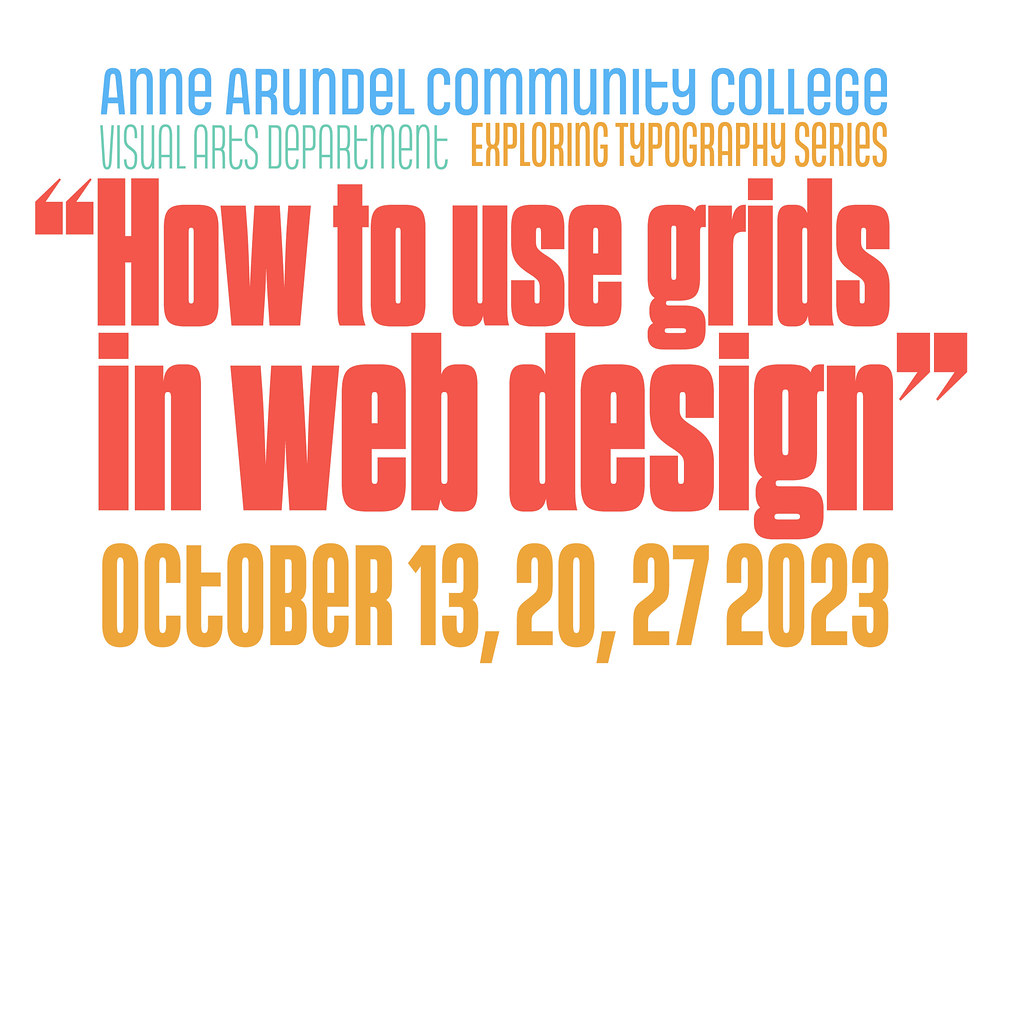This image is a promotional flyer set against a white background. At the very top, in light blue lettering, it reads "Anne Arundel Community College." Directly below, in light green, it states "Visual Arts Department." Continuing from the center to the right edge in light gold or yellow, it announces the "Exploring Typography Series." The prominent and bold feature of the flyer is the bright red, large, sans-serif text that spans two lines, reading "How to Use Grids" on the first line and "In Web Design" on the second line. Lastly, at the bottom of the flyer, in the same light gold or yellow text, are the dates "October 13, 20, 27, 2023." There are no graphical elements in the image, only varied text colors and sizes to draw attention to key information.